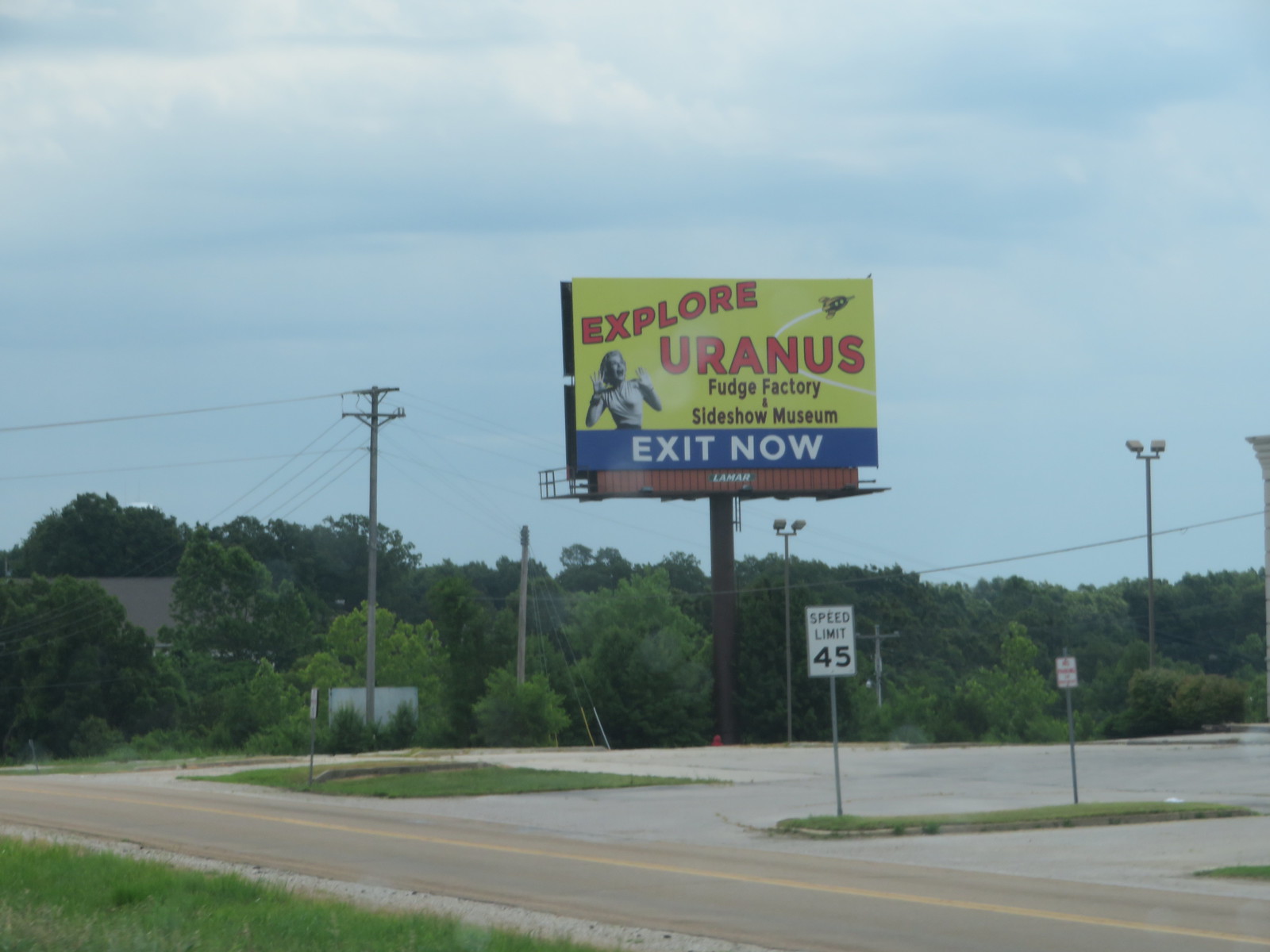The image features a large billboard mounted on a tall post, prominently situated near a roadway. The billboard has a vibrant yellow background with bold red letters that read "EXPLORE URANUS." Positioned beneath this text are the phrases "FUDGE FACTORY" and "SIDESHOW MUSEUM" in clear black letters. The focal point of the advertisement is a woman with her hands raised in the air and a shocked expression, emphasizing the quirky and amusing nature of the attractions mentioned.

Below the primary message, the billboard has a blue section with the directive "EXIT NOW" in white font, guiding travelers to the nearby exit. In the foreground, the road stretches out, marked by a yellow divider line. To the left, there is a stretch of grassy area, while a "SPEED LIMIT 45" sign is clearly visible.

In the background, the scenery includes a cluster of trees, giving way to what appears to be a large parking lot on the right. The overcast sky is filled with a mix of gray and white clouds, creating a moody atmosphere. Numerous telephone poles and streetlights are also seen lining the horizon, adding to the detailed elements of the scene.